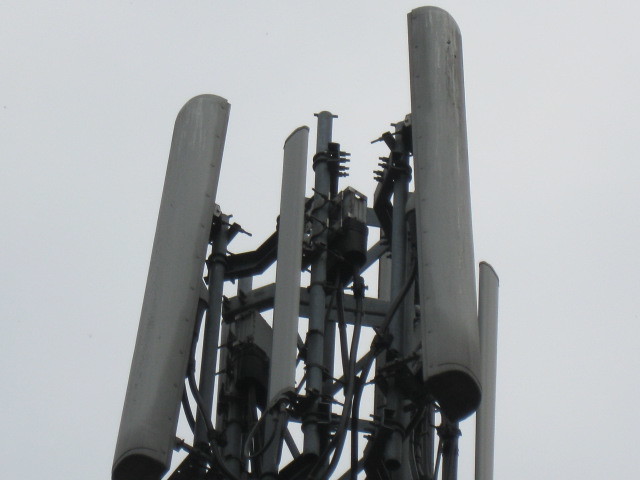This is a detailed black-and-white photograph of the upper section of a cellular tower. The central structure is composed of robust steel posts connected by crossbars, creating a rectangular frame that spans the entire height of the visible structure. Numerous large, shielded antennas, characterized by their cylindrical, white metal plating, are mounted at the top. Additionally, there are multiple vertical gray metal poles running from the bottom to the top of the image. These poles support and are interspersed with a network of substantial electrical cables, screws, and various fixings. Semi-circular, white half-cylinder objects, probably additional antenna elements, are vertically positioned on either side of the poles, along with several metal bars extending horizontally across the structure. The background is a bleak, gray sky, which accentuates the stark, complex, and somewhat hazardous appearance of this towering, spiky array of equipment.